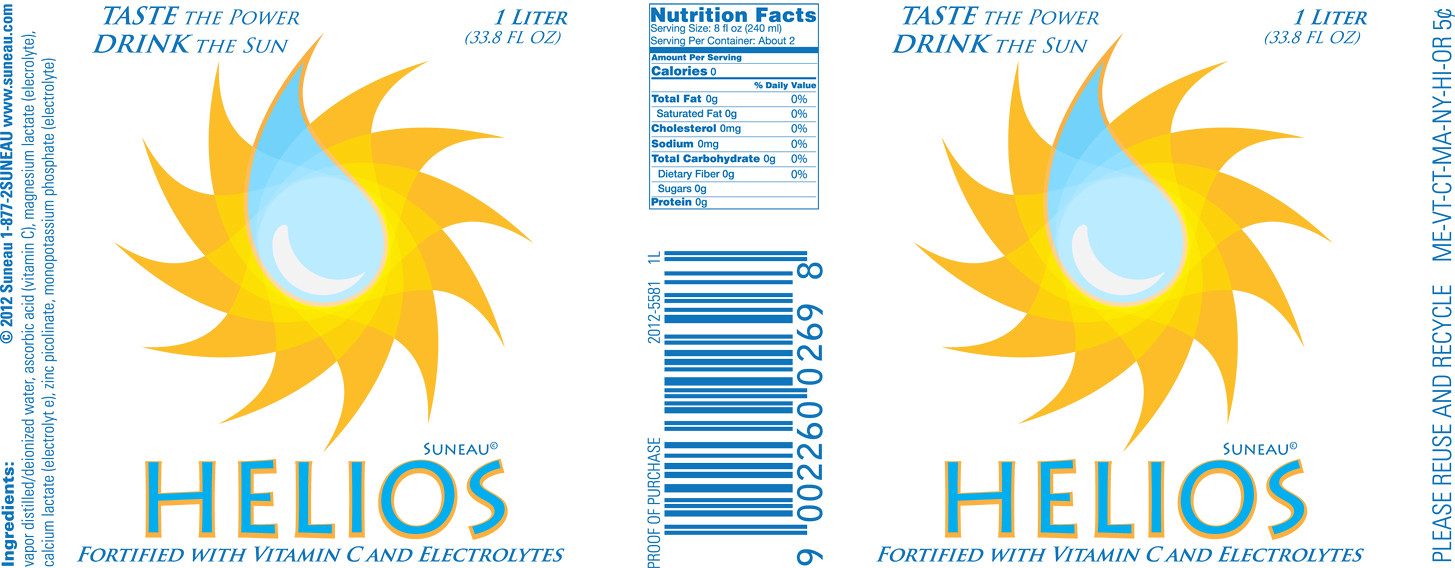This color image depicts an unfolded drink carton, laid out to showcase its entirety. The front and back panels of the carton are identical, positioned on the left and right sides of the image. The middle section, representing what would be the side of the carton, features a barcode at the bottom and a nutritional facts label at the top, detailing the carbohydrate, fat, and other nutrient contents.

Set against a white background, the carton prominently displays the brand name "Helios," accompanied by the tagline "Fortified with Vitamin C and Electrolytes." Central to the design is a spiraling sun emblem, with curved rays extending in a clockwise pattern, centered around a large, vivid blue water droplet.

At the top of the carton, one side reads "Taste the Power, Drink the Sun," while the opposite side indicates the product volume as "One Litre." Additional text is also visible running along the edges of the carton, providing more details about the product.